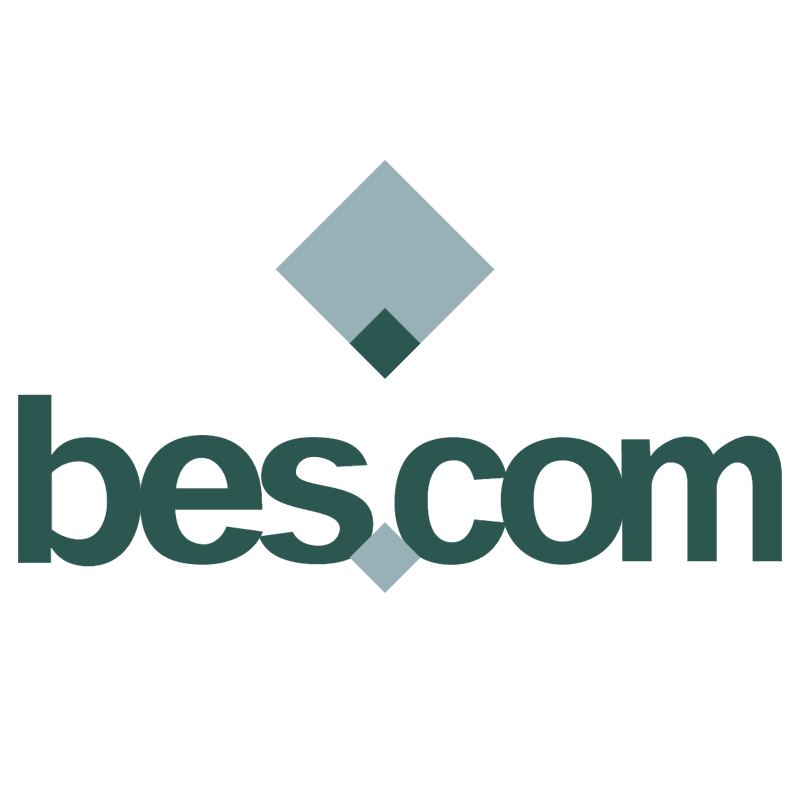The image features the logo for the company best.com, spelled entirely in lowercase letters. The text "B-E-S" and "C-O-M" are rendered in dark green, with the letters slightly touching each other: B and E, S and C, C and O, and O and M are all connected, while E and S are not. The period in the domain name is depicted as a light gray dot. Above the text, centrally positioned between the 'S' in "best" and the 'C' in "com," is a larger gray triangle. This triangle has a small dark green triangle occupying its bottom corner. The entire logo is set against a clean white background.